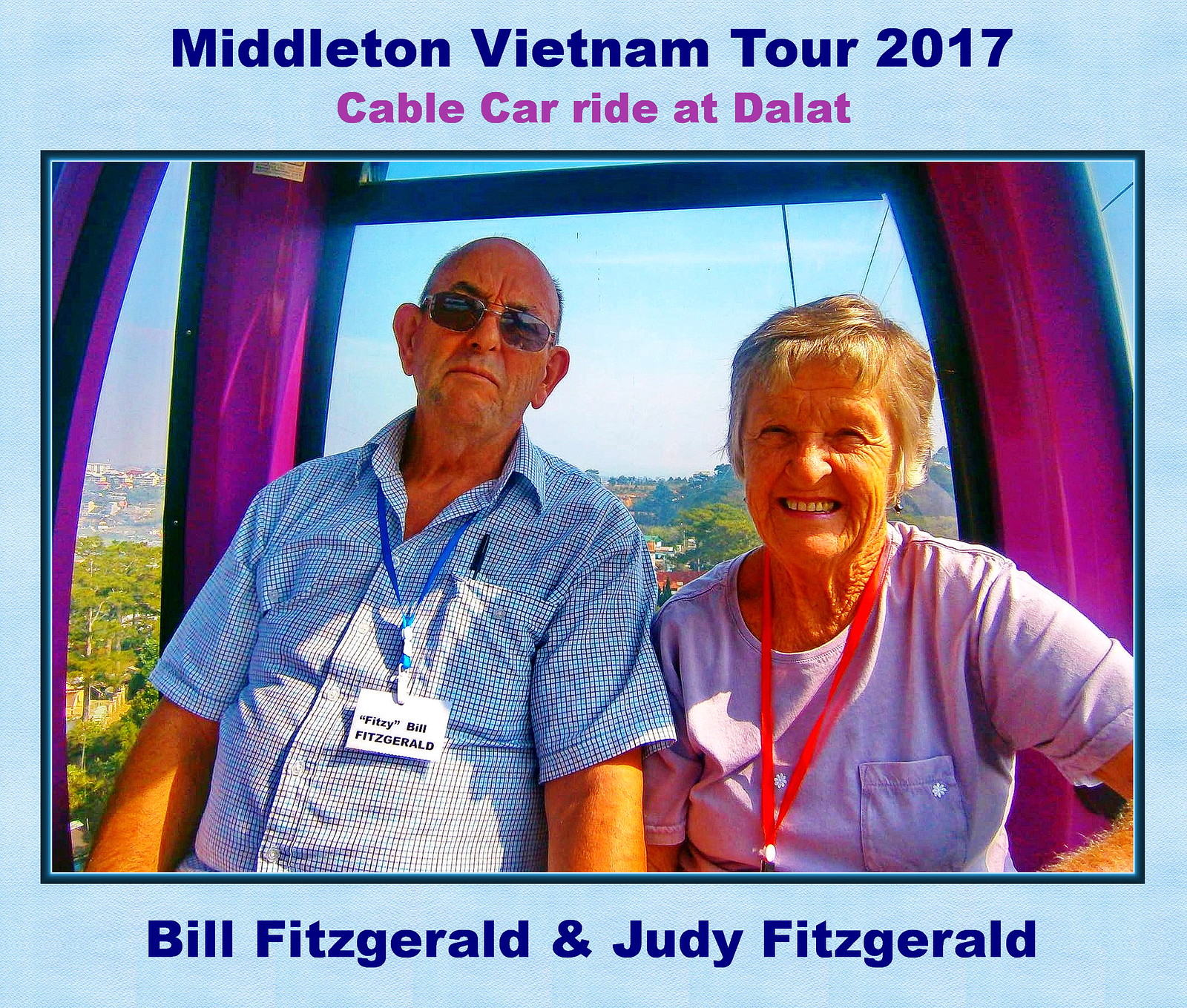The image is a rectangular, horizontal photograph with a light blue border. At the top, in dark letters, it reads "Middleton Vietnam Tour 2017," followed by "Cable Car Ride at Dalat" in red or purple letters. Below the photograph, in blue letters, it says "Bill Fitzgerald and Judy Fitzgerald." The central photo features an older man and woman, likely in their 70s, identified as Bill and Judy Fitzgerald. Both are wearing name tags around their necks. Bill, who is minimally haired and wearing sunglasses, is dressed in a light blue shirt with a pencil in his pocket. Judy, with light brown hair and a big smile, is dressed in a purple t-shirt and her name tag has a red rope. The couple is seated in a bright pink, some captions mentioning purple, cable car, with a clear view of the city skyline below them and a backdrop of clear blue skies. Both appear to be enjoying their trip, with Judy expressing more visible happiness than Bill.